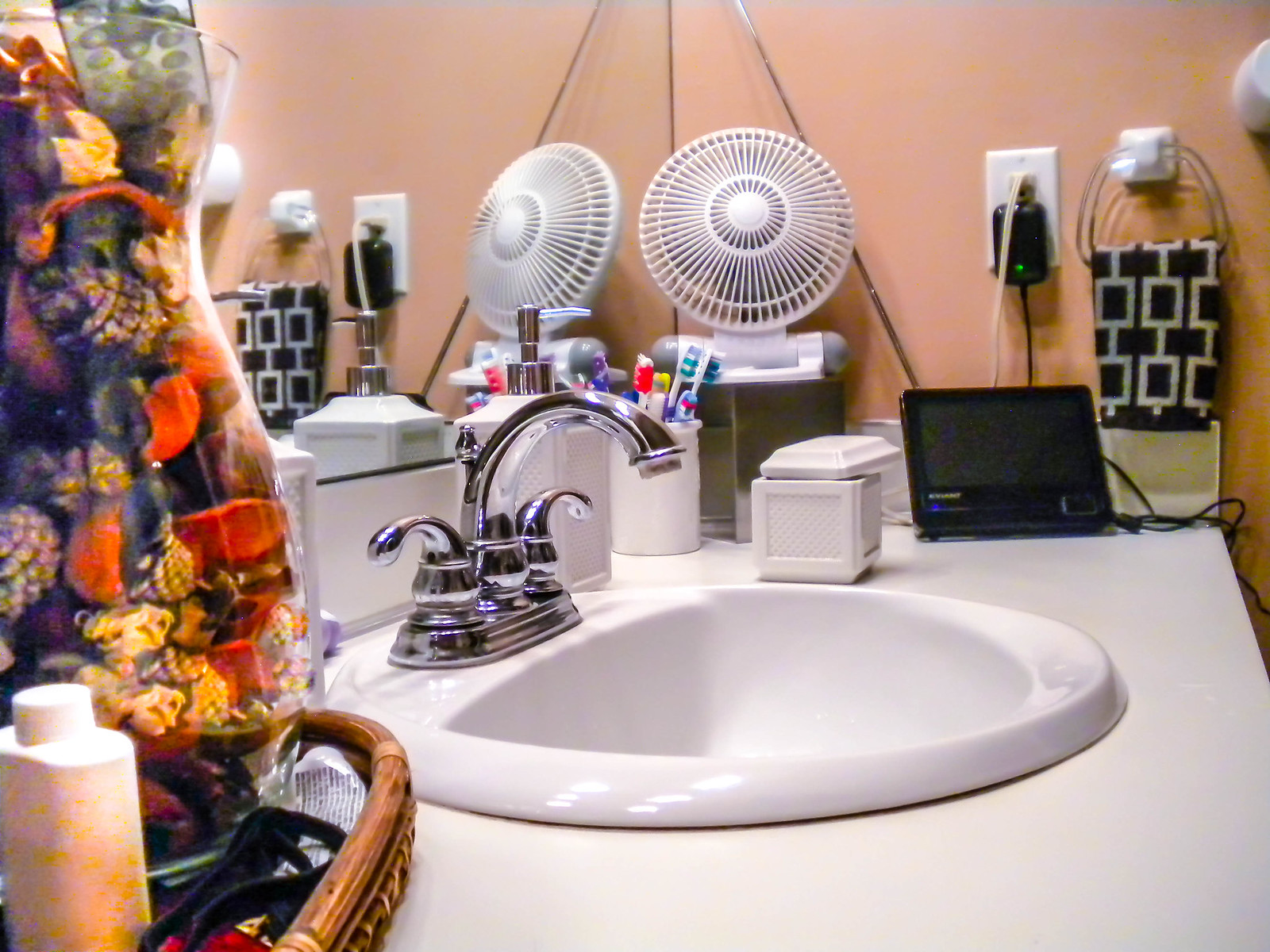This close-up image captures a detailed view of a bathroom counter brimming with various items. To the far right, a white mini-fan sits elevated on a small platform. Adjacent to the fan is a device resembling a radio or a small-screen gadget. Moving leftward, a small white ceramic box adds to the collection of countertop items. A wall outlet is visible, with two cords plugged in, underlining the functionality of the space. 

On the wall, a white hook holds a neatly folded face cloth, poised for use. The centerpiece of the sink area is a white ceramic basin paired with a sleek metal faucet. Behind the sink, a large mirror reflects the setting, enhancing the sense of space. Complementing the mirror is an elegant glass vase filled with assorted pine cones, dried flowers, and potpourri, adding a touch of natural décor. Curiously, a remote control protrudes from the top of this vase.

In front of the vase, a small basket houses various toiletries, including a partially obscured white bottle, its exact contents indiscernible due to the peculiar lighting and angle of the shot. This intricate arrangement of everyday bathroom items provides a glimpse into a meticulously organized yet lived-in space.